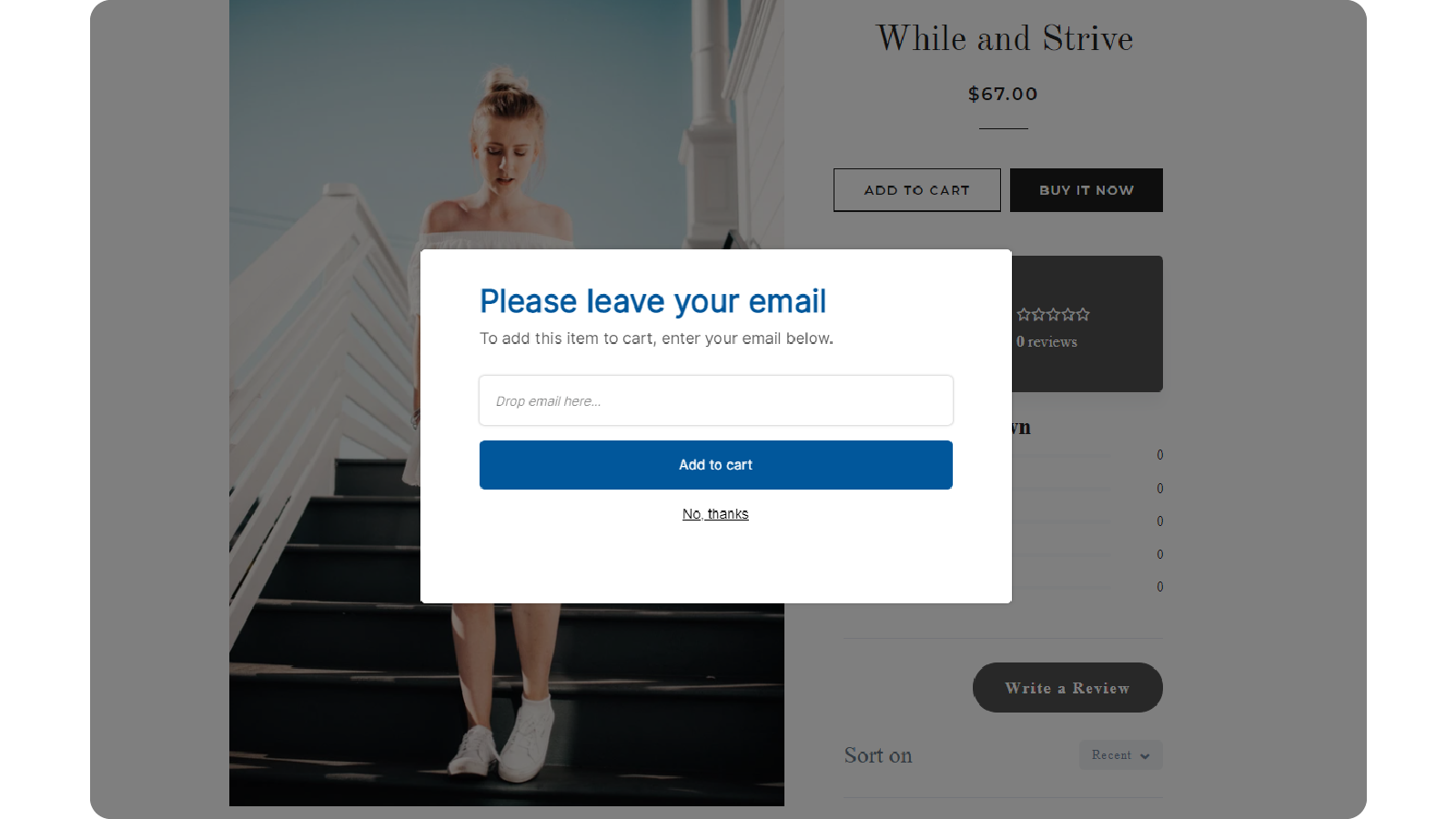A detailed photographic image of a webpage displays a pop-up in the foreground, causing the rest of the webpage to fade to a grayish tone. The pop-up is a bright white rectangular box that prominently features a request in blue text: "Please leave your email." Below this, in black text, it instructs users, "To add this item to cart, enter your email below." There are two interactive elements on the pop-up: a white rectangular button labeled "Drop email here" and a blue button reading "Add to Cart." Additionally, an underlined black text option says "No thanks."

In the background of the image, the webpage content is partially visible. It features a photograph of a woman wearing a white dress and white tennis shoes, descending a staircase with white railings against a blue sky backdrop. Accompanying this image, the product information is displayed: it reads "White Dress - Strive for $67," followed by buttons labeled "Add to Cart" and "Buy It Now." The product currently has zero reviews, and there is a gray button at the bottom of the webpage prompting users to "Write a Review."